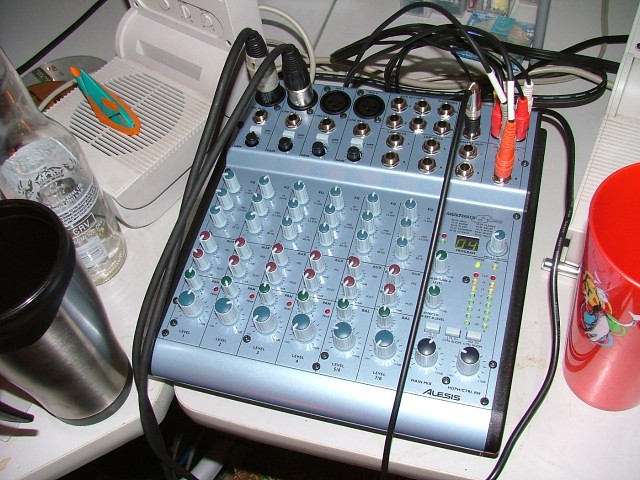The image portrays a baby blue circuit board or control panel, covered with numerous multi-colored knobs and dials arranged in rows. Of the knobs, red, green, light blue, and dark blue or black are visible. The top section of the device is densely populated with various cords plugged in, some with orange-tipped connectors, reminiscent of auxiliary cords used in old television or audio equipment. Black cords with silver tips are also attached to the upper left corner. The board, potentially a sound control device or part of medical or laboratory equipment, has several rows of eight lights or buttons across its surface. It sits on a white table, surrounded by a silver and black thermos, an empty bottle resembling a Corona beer bottle to the left, and a red cup with a colorful design featuring yellow, green, blue, and white on the right. The setting could be a hospital, laboratory, or studio. Notably, no people are present in the image.